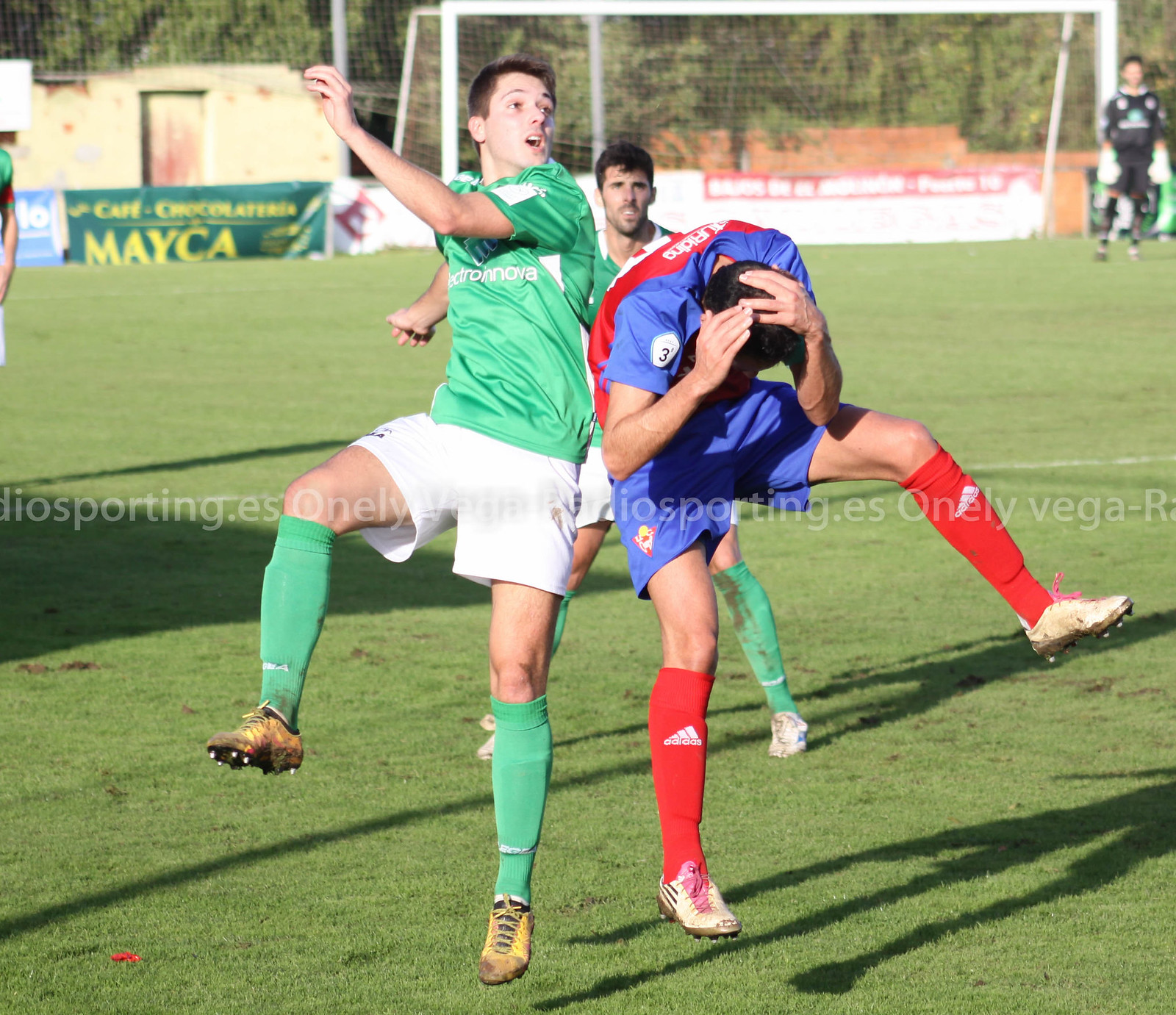The image captures an intense moment in a soccer game with a close-up of three airborne players in action on a sunny soccer field. The player on the left is wearing a green jersey, white shorts, long green socks, and yellow cleats; he's jumping, seemingly trying to head the ball. To his right, another player in a blue jersey, blue shorts, long red socks, and light yellow cleats is also midair with his hands over his head, possibly shielding himself. Behind them, a third player in a green jersey, green socks, and white cleats watches the action unfold. In the background, there is a soccer goal and banners with various advertisements, including one partly obscured watermark in gray text reading "IOSPORTING.ES" across the image. A fourth individual, presumably the goalie, dressed in all black, is visible in the distance, observing the scene. The weather appears to be warm and clear, making for a perfect day for soccer. The setting is bustling with activity, indicative of a competitive male soccer match.